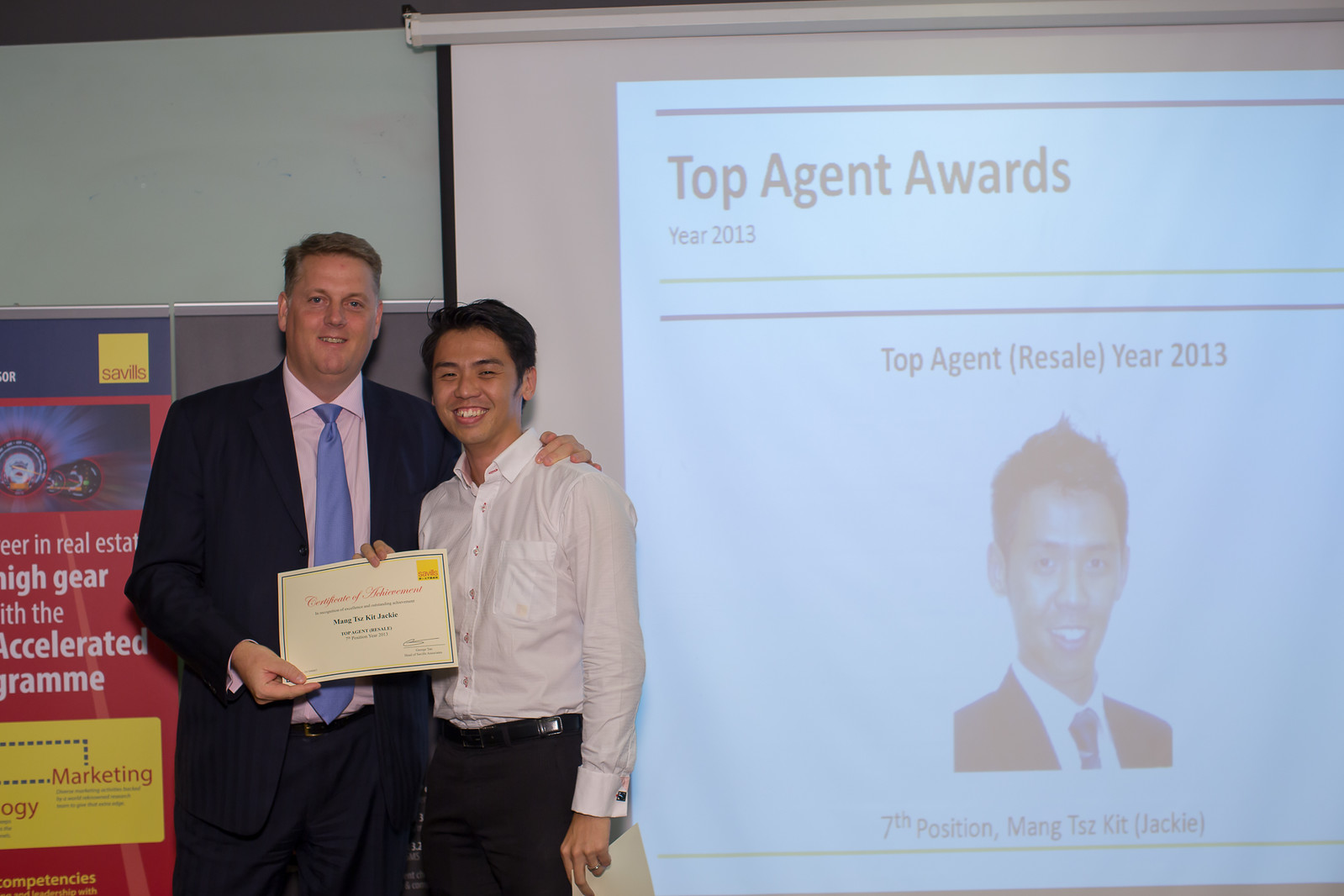In this indoor photograph, we observe an award ceremony featuring two men positioned towards the left side of the image. The man on the left, who is Caucasian and slightly heavyset, is dressed in a black suit with a white shirt and a light blue tie, while the man on the right, identified as Mang Sukit (Jackie), dons black pants with a black belt and a white button-down shirt without a tie. Both are smiling and holding up a certificate together. The backdrop includes several posters and notable text projected on a screen to the right. The projection boasts the title "Top Agent Awards Year 2013" and "Top Agent Resale Year 2013," indicating that Jackie secured the "7th Position." The screen also features Jackie's photograph. The color palette of the image includes shades of black, gray, blue, red, yellow, tan, and light blue.